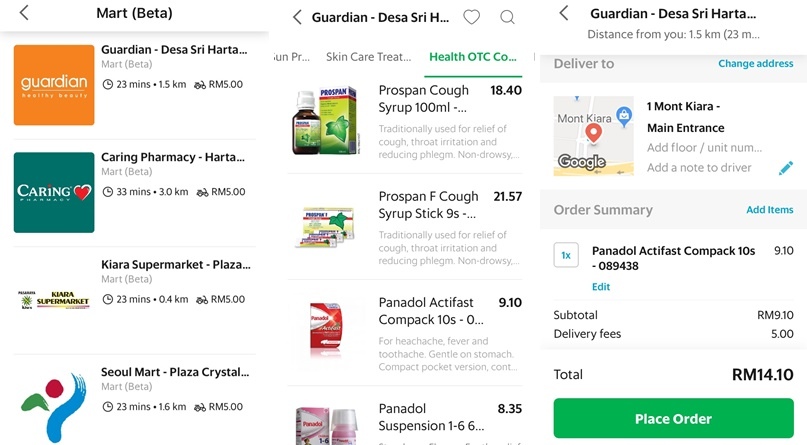The image features a detailed list against a white background. On the left side, it is marked with "Beta" in parentheses. Below that, there's a gray horizontal line followed by a series of store names and their distance from a specified point. The list includes:

1. "Guardian Desert Sri Harta" with an orange square labeled "Guardian" next to it, indicating a distance of "23 minutes, 1.5 KM, ring.co".
2. "Caring Pharmacy" showing a distance of "33 minutes, 3.0 KM".
3. "Kiara Supermarket Plaza" marked with a distance of "23 minutes, 0.4 KM".
4. "Soul Mart Palato Crystal" listed with a distance of "23 minutes, 1.6 KM".

On the right side of the image, there is a depiction of two products: a box of cough syrup and a bottle of cough syrup. The text alongside these items describes:

1. "ProSpan Cough Syrup 100ml" priced at "18.40".
2. "ProSpan F Cough Syrup Stick 9" priced at "21.57".
3. "Panadol ActiFast Compact 10S" priced at "9.10".
4. Additionally, it mentions "Panadol Suspension".

The image provides a clear and organized list of pharmacies and nearby supermarkets along with the display of specific medical products and their prices.